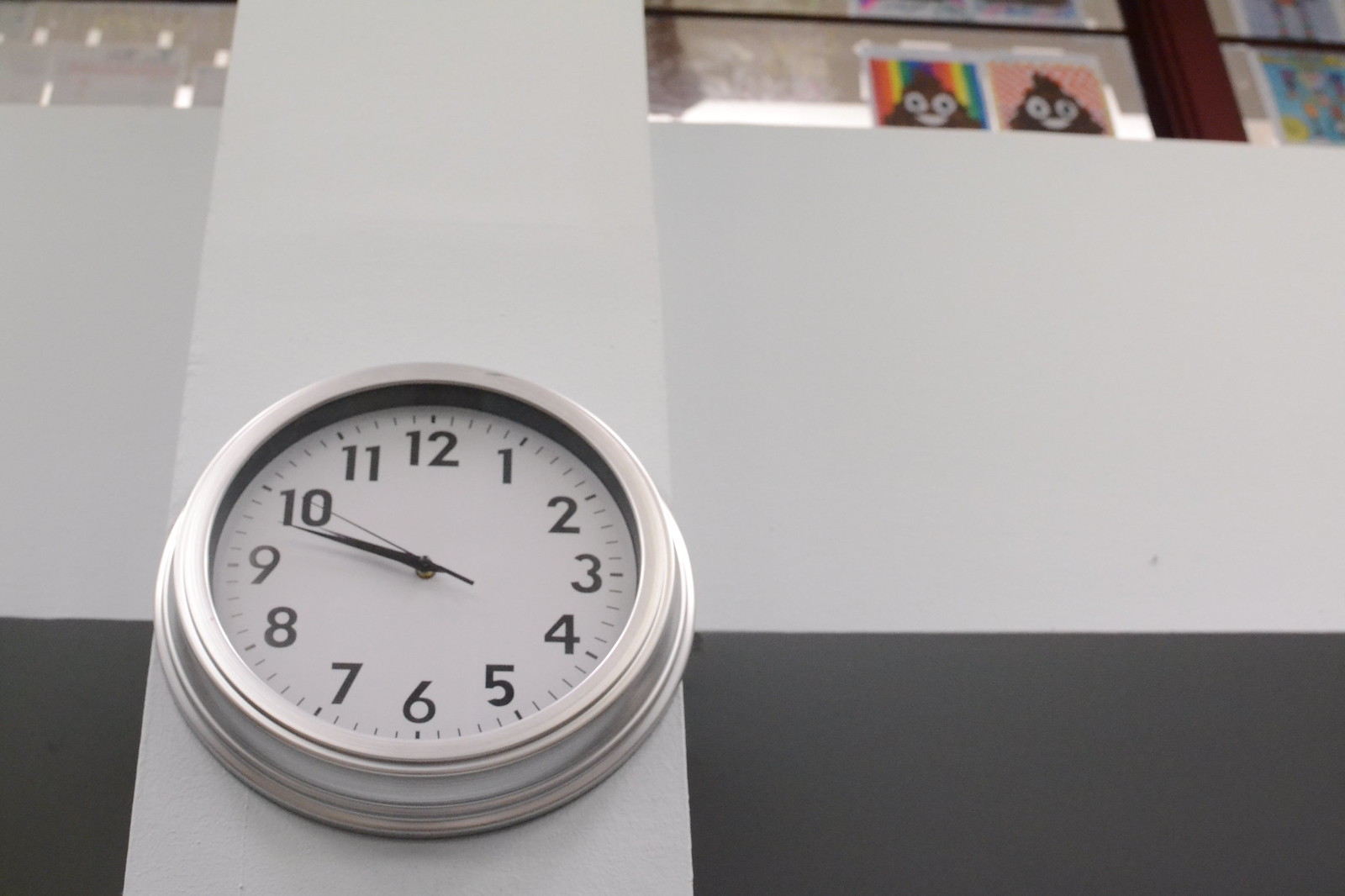The image depicts a simple, round clock with a stainless steel-colored rim and a white face featuring standard black numerals and a red second hand. The clock reads approximately 12 minutes to 10 and is mounted on a white support beam between the first and second floors of a building. The wall behind it is decorated with thick horizontal bands of gray and shades of off-white. Above the clock, there are windows with a shelf or sill displaying children's drawings. Two drawings prominently feature printed poop emojis, each with different backgrounds—one with a rainbow design and the other with a pink design. To the left of the clock, there is a reflection of light, adding a bit of ambiance to the scene, which appears to be in a school building or similar setting.